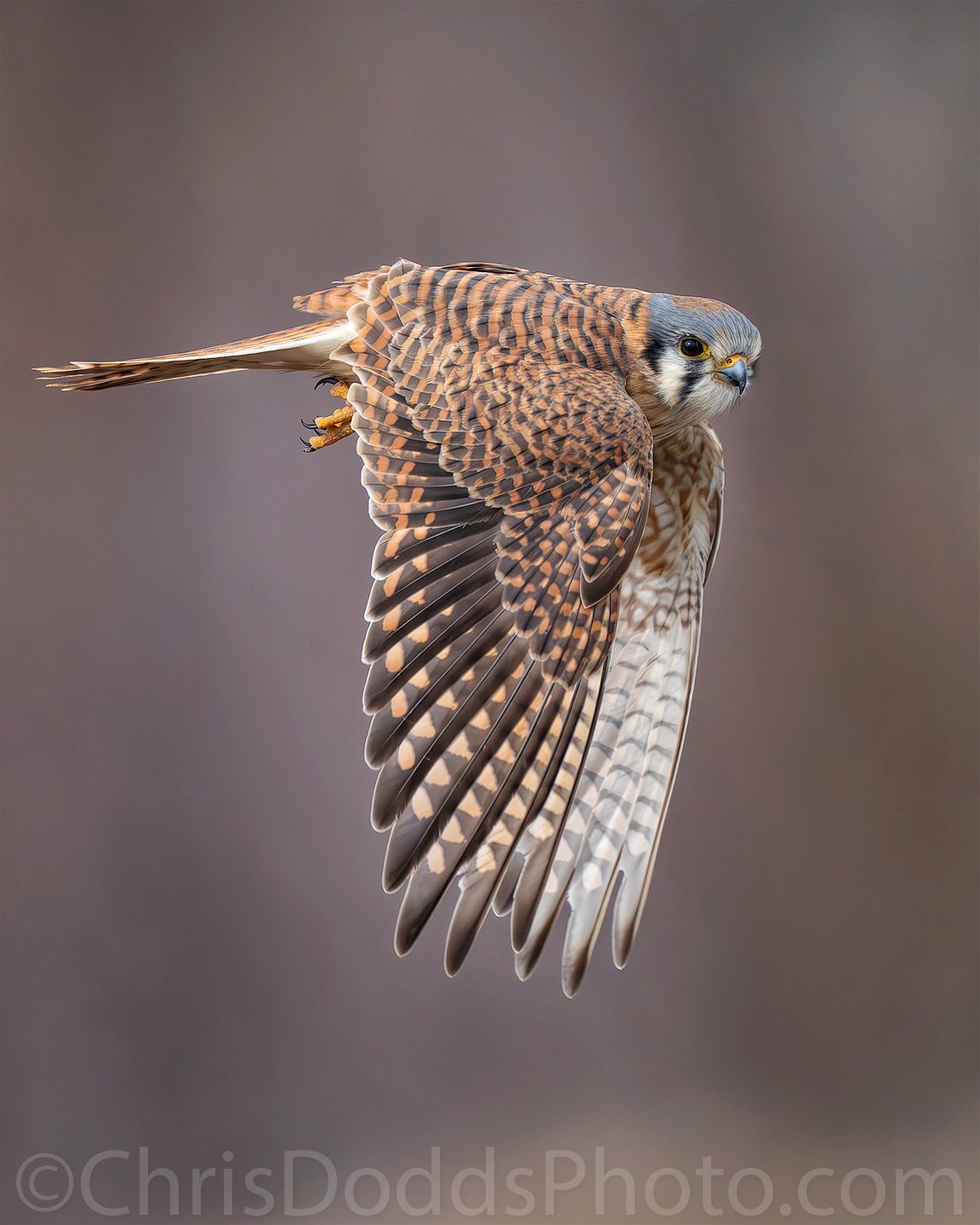In this color photograph by Chris Dodds (chrisdoddsphoto.com), a bird, possibly a falcon or heron, is captured in mid-flight, flying from left to right with its wings in a fully downturned position. Centered in the image against a grayish, bokeh-effect background, the bird displays a striking color pattern. The head is predominantly grayish-blue with a distinctive black dot and white markings under the eye and beak. The beak itself is black with a yellow patch where it meets the face. The bird's body feathers exhibit an intricate mix of black and brown, while the undersides show white with black lines and pointy shapes. Its partially visible tail appears brown on top and white underneath. The legs, stretched back under its body, are a vivid orange with black claws. The copyright notice "Chris Dodds Photo" is clearly visible at the bottom of the image.